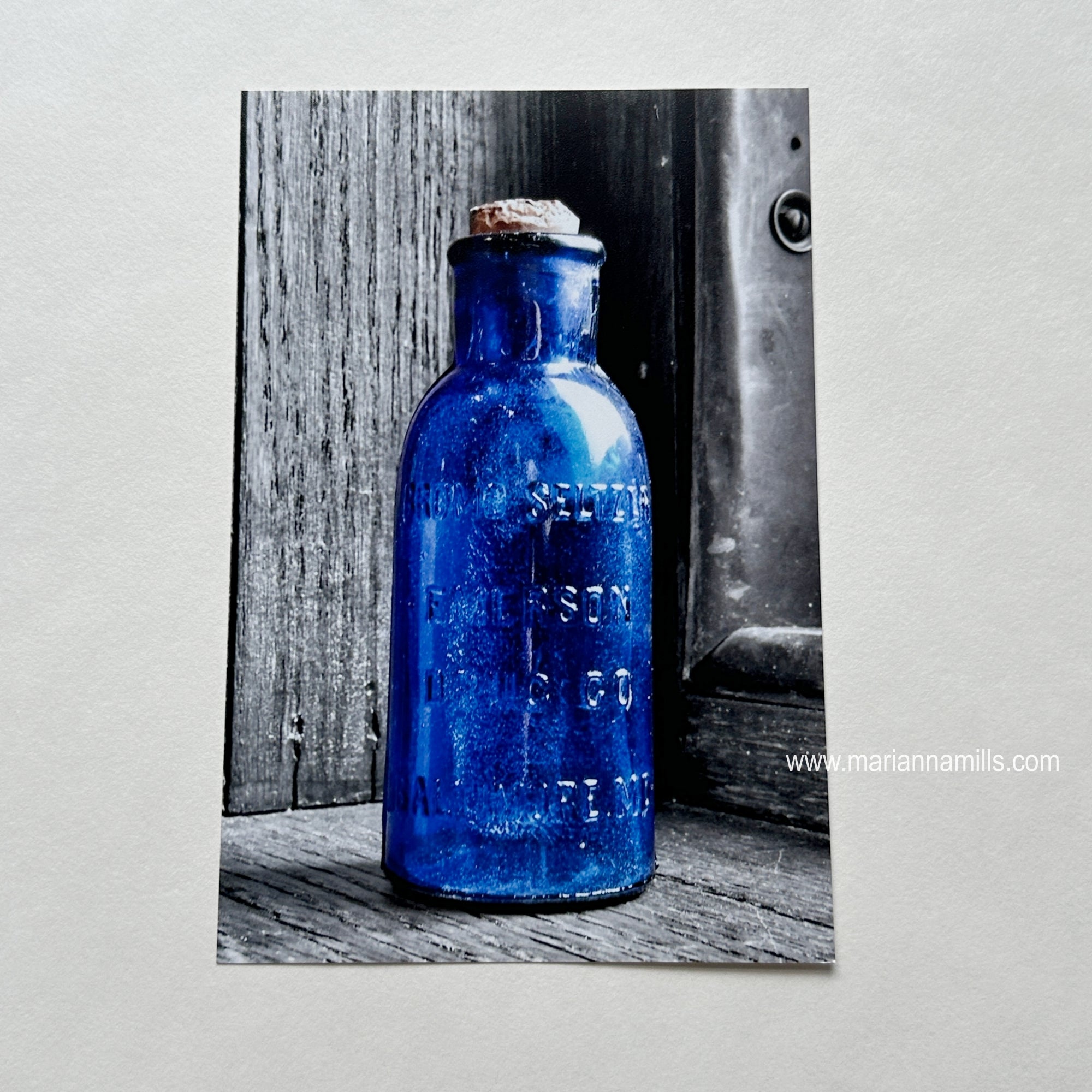This photograph, presented within a light gray background, showcases a captivating blue glass bottle with an aged, distressed cork. The background, evocative of an antique black-and-white film, accentuates the vivid blue of the bottle, which is ornately engraved with unreadable raised lettering. The bottle, appearing to be an antique due to its thick glass and worn cork, stands prominently on a weathered wooden surface against a similarly aged wooden backdrop. A piece of metal with a bolt is visible in the right corner, adding to the rustic charm. The image has a noticeable border, and at the bottom right, the photographer's website, www.marianamills.com, is clearly inscribed.